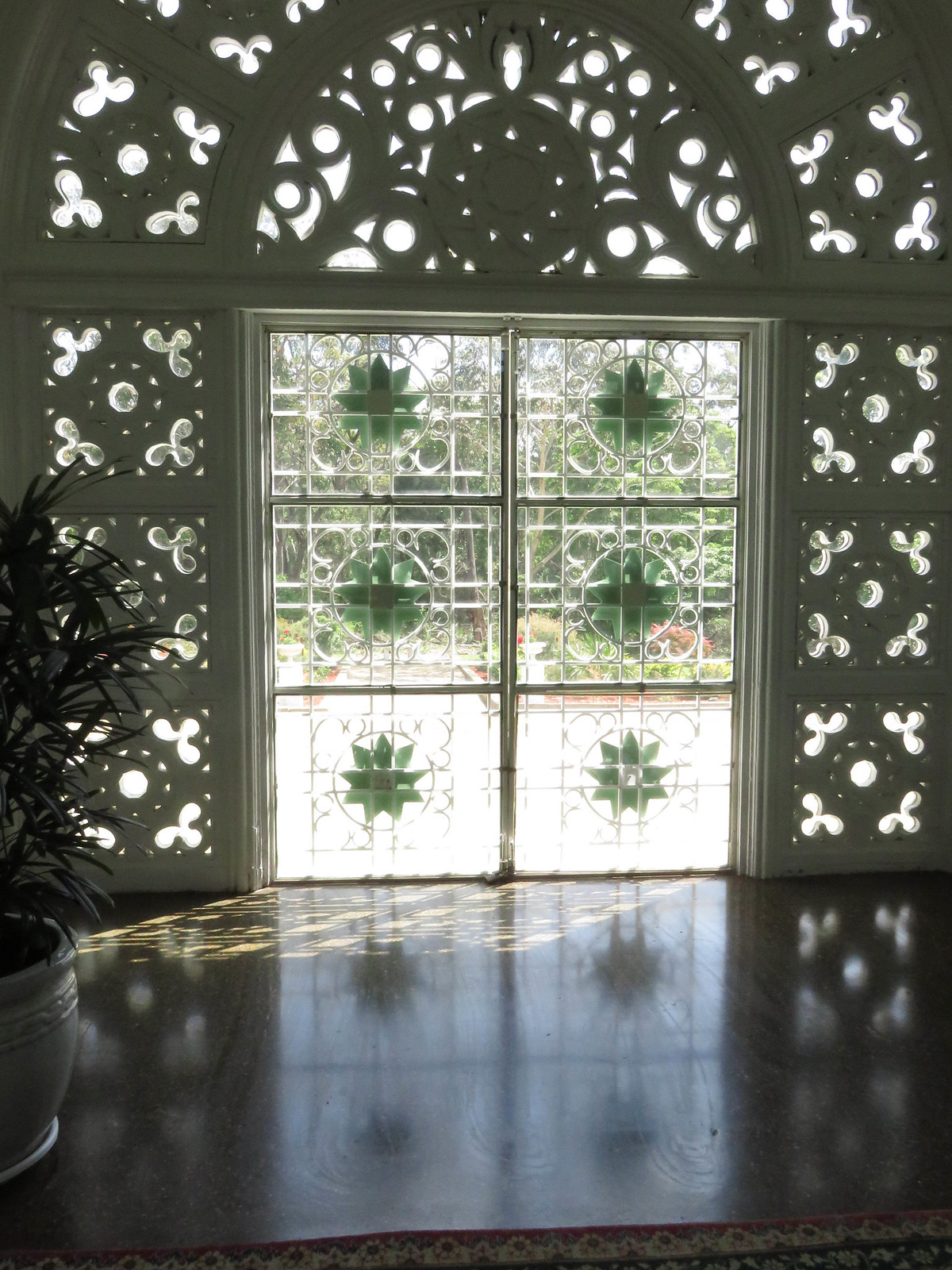The photograph depicts the interior of a building focusing on a large, ornate door or window made of white concrete. This door, with its six paneled design, features three large panes of glass per door, each adorned with a green stained glass nine-point star at the center. Light streams through these unique cutouts, casting intricate shadows and reflections on the sleek, hard floor—likely marble or concrete. To the left, partially cut off, sits a white potted plant. A long carpet extends from the foreground, contrasting with the otherwise bare and glossy floor. The exterior backdrop showcases vivid green plants or trees illuminated by a soft yellowish-white light filtering through the windows, enhancing the bright and airy ambience of the scene.